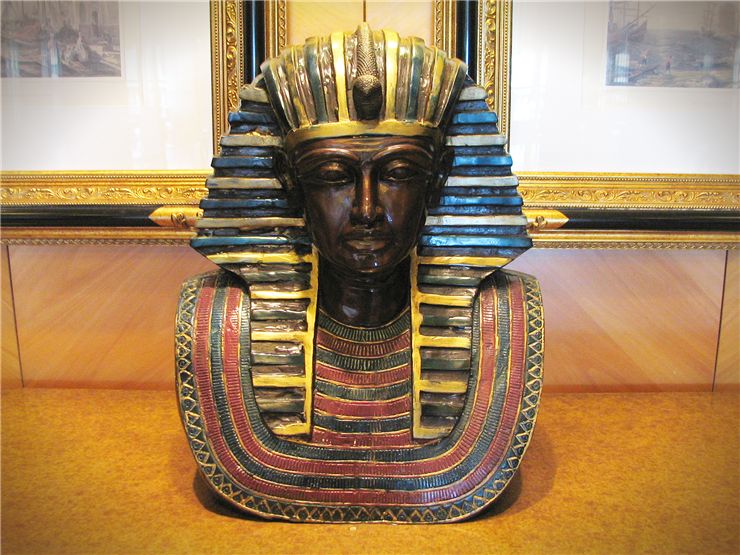In a museum setting dedicated to Egyptian artifacts, there stands a grand bust of an Egyptian pharaoh, reminiscent of King Tut. The pharaoh's face is a rich dark brown, with open, striking brown eyes. He is adorned with the iconic nemes headdress, featuring a serpent at its center, symbolizing protection and royalty. The headdress displays intricate stripes of gold, black, blue, and white cascading down towards the chest. The pharaoh also dons a resplendent broad collar characterized by hues of red, blue, black, and gold, adorned with a zigzag pattern along its edges. This imposing figure is positioned on a yellow flooring, with a sumptuous gold-wrought frame partly visible behind its head, flanked by two slightly blurred pictures on the walls. The overall focus of the scene is undeniably on this magnificent representation of ancient Egyptian royalty.